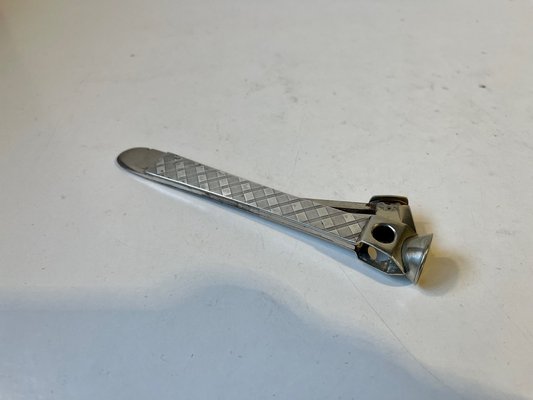In the image, there is a broken metallic object that may have been a hair clip or a tie clip. This clip is made of silver metal and exhibits a designed pattern on the front, consisting of diagonal box shapes. The clip includes an attachment with a large hole in the metal and a cup-shaped protrusion towards the front. Beneath this main piece, there's another metallic component that may serve as the backing necessary for the clip’s function. The item is placed on a slightly dirty white background. The object also has shadows, adding depth to the image. The entire thing resembles a metallic contraption, and while difficult to precisely identify, its intricate details suggest it was once a functional accessory.